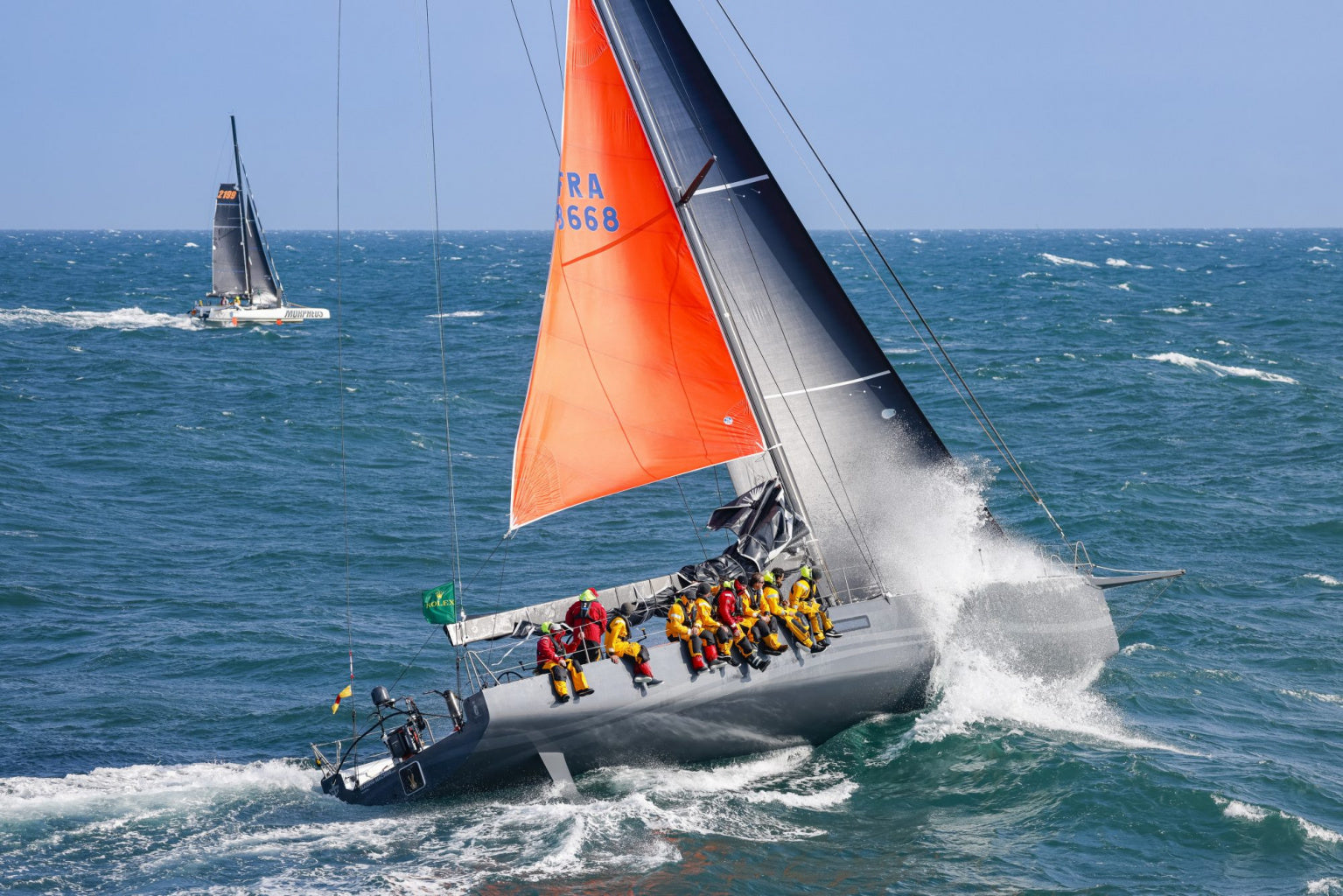The image is a vivid color photograph of a sailboat navigating the ocean under a clear blue sky. The boat, which seems designed for a race, is equipped with a large orange sail marked with "RA 668" in blue, and a gray sail. It has a grayish body. The sea around the boat is choppy, creating white foam as the vessel moves through the water. Several people wearing water-resistant yellow and red suits are positioned at the edge, leaning to one side to balance the boat as it appears to make a turn. In the background, another sailboat with a white body and gray sails is visible, similarly surrounded by the blue, sunlit water.